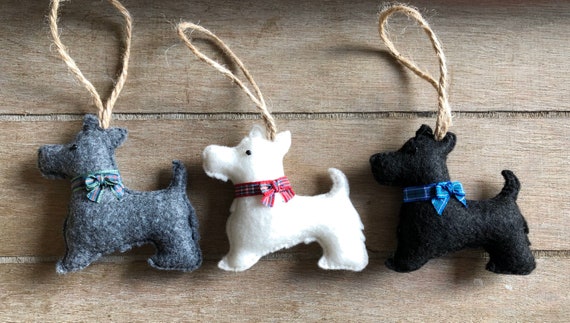The image features three small, handmade cloth Christmas ornaments in the shape of terrier dogs, each with a loop of hemp or jute twine for hanging. The scene is set on an unstained, raw plywood floor, with the camera capturing the view from directly above in landscape mode. The dogs are identical in size and shape, each with black eyes and looking to the left. From left to right, the first dog is gray with a green and red plaid bow, the middle dog is white with a gray and red plaid bow, and the rightmost dog is black with a blue, purple, and green plaid bow. Each ornament has a light twine loop extending from the top, showcasing their purpose as hangable decorations.